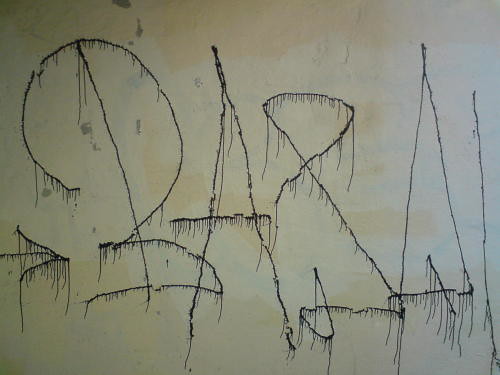The image depicts a piece of graffiti or art on a white wall that has patches of gray and tan, likely from previous attempts to cover other graffiti. The artwork features thin black lines that are not straight but slightly curved, with noticeable paint drips along each line. On the left side of the image, there is a black arrow pointing to the right. Following the arrow is either a letter 'D' or the number '2' due to its ambiguous shape, which is immediately succeeded by a letter 'A' resembling a witch hat. There appear to be other symbols including a debatable 'B' and 'P', forming what might be interpreted as "BAP". Towards the right end of the wall, there's a triangle and a few squiggly lines beneath it. These elements give the impression of a creative, yet chaotic, urban artwork.